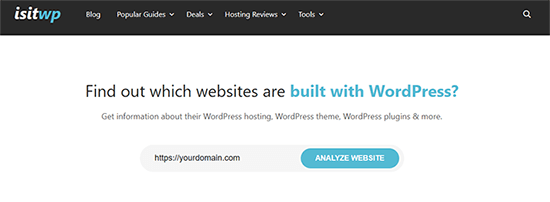This screenshot captures a section of a website, mimicking the dimensions of a desktop or laptop display. The absence of borders on the sides and bottom makes it seamlessly blend into the background, while a nearly black header at the top runs the full width of the page, demarcating the site's boundary.

In the upper left corner of this header, the website's name or its abbreviation appears as "isitwp," written in continuous lowercase letters. The "isit" portion is in white text, while "wp" is rendered in blue. To the right of this logo, several clickable text links are arranged horizontally. These links include options such as "Blog," "Popular Guides," "Deals," "Hosting Reviews," and "Tools." On the far right side of the header is a magnifying glass icon, indicating a search functionality.

Directly beneath the header, a white background section features a prominent query: "Find out which websites are built with WordPress? Get information about their WordPress hosting, WordPress theme, WordPress plugins, and more." This text invites users to engage with the site's main function. Below this text, there is a URL input box accompanied by a blue "Analyze Website" button, offering an interactive tool for users to analyze the specified website.